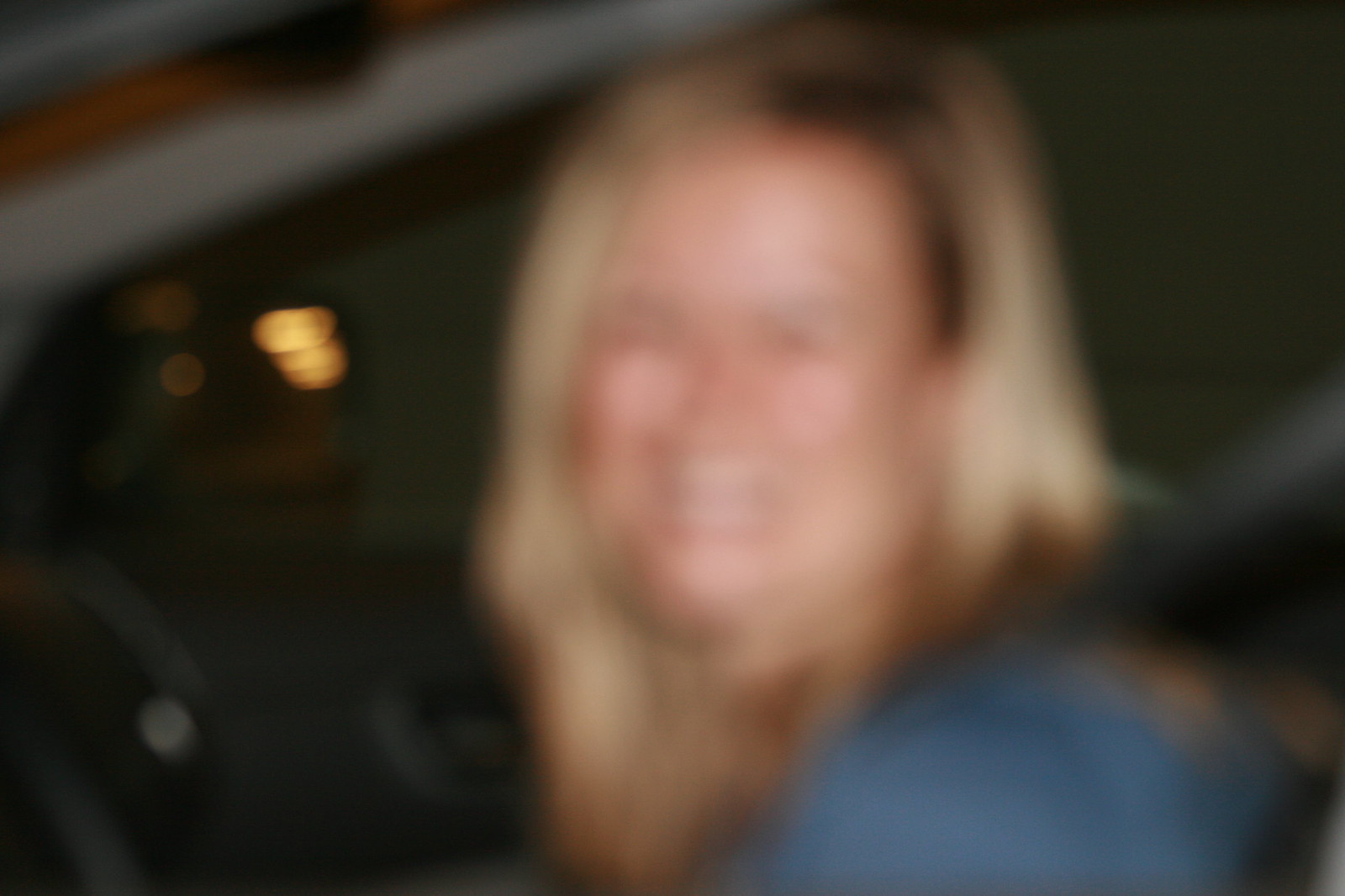A blurred photograph captures a Caucasian woman with long blonde hair, seated inside a car. She is smiling warmly and wearing a blue top. Despite the blurriness, it is evident that she is secured by a seatbelt. The car's interior, including dark door paneling and some front features, is partially visible. The image also includes the reflection of a camera flash on the window. The woman's placement suggests she might be in either the driver's or passenger's seat.